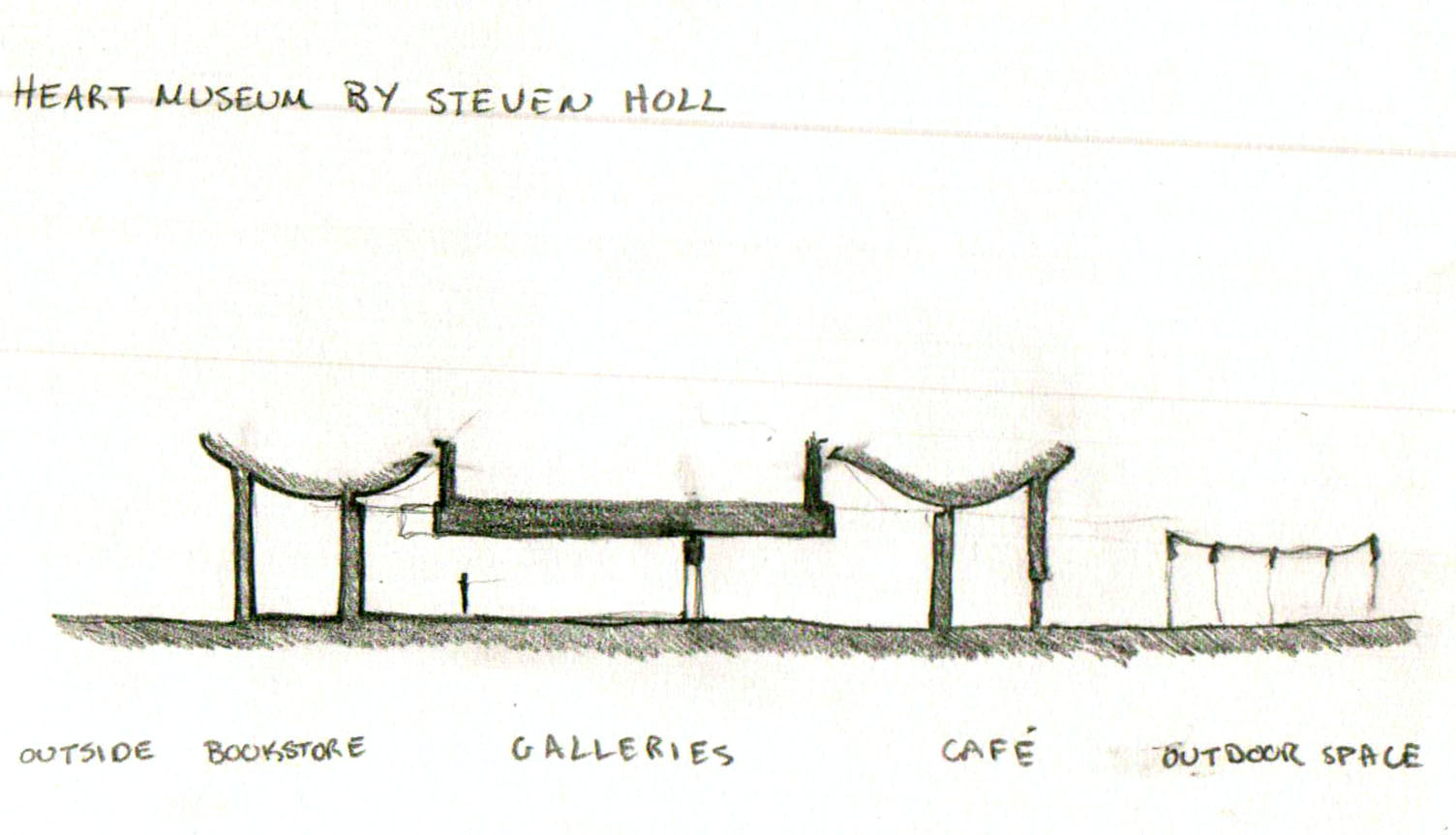The image is a detailed black-and-white drawing titled "Heart Museum by Stephen Hull," as written in pencil in the upper left-hand corner. The composition features a flat, low structure with a uniquely indented roof that rises higher on the sides and is flat in the middle. Prominent in the scene are two large, curving beams that form a half-circle shape with a dark, rectangular bar hanging between them. This structure appears to possibly support a swing or another element of the museum. To the right, there are more vertical lines that resemble distant power lines, all sketched in a graphite pencil style. At the bottom of the drawing, separated by gaps, are the words: "outside," "bookstore," "galleries," "cafe," and "outdoor space," suggesting the different planned sections of the Heart Museum.